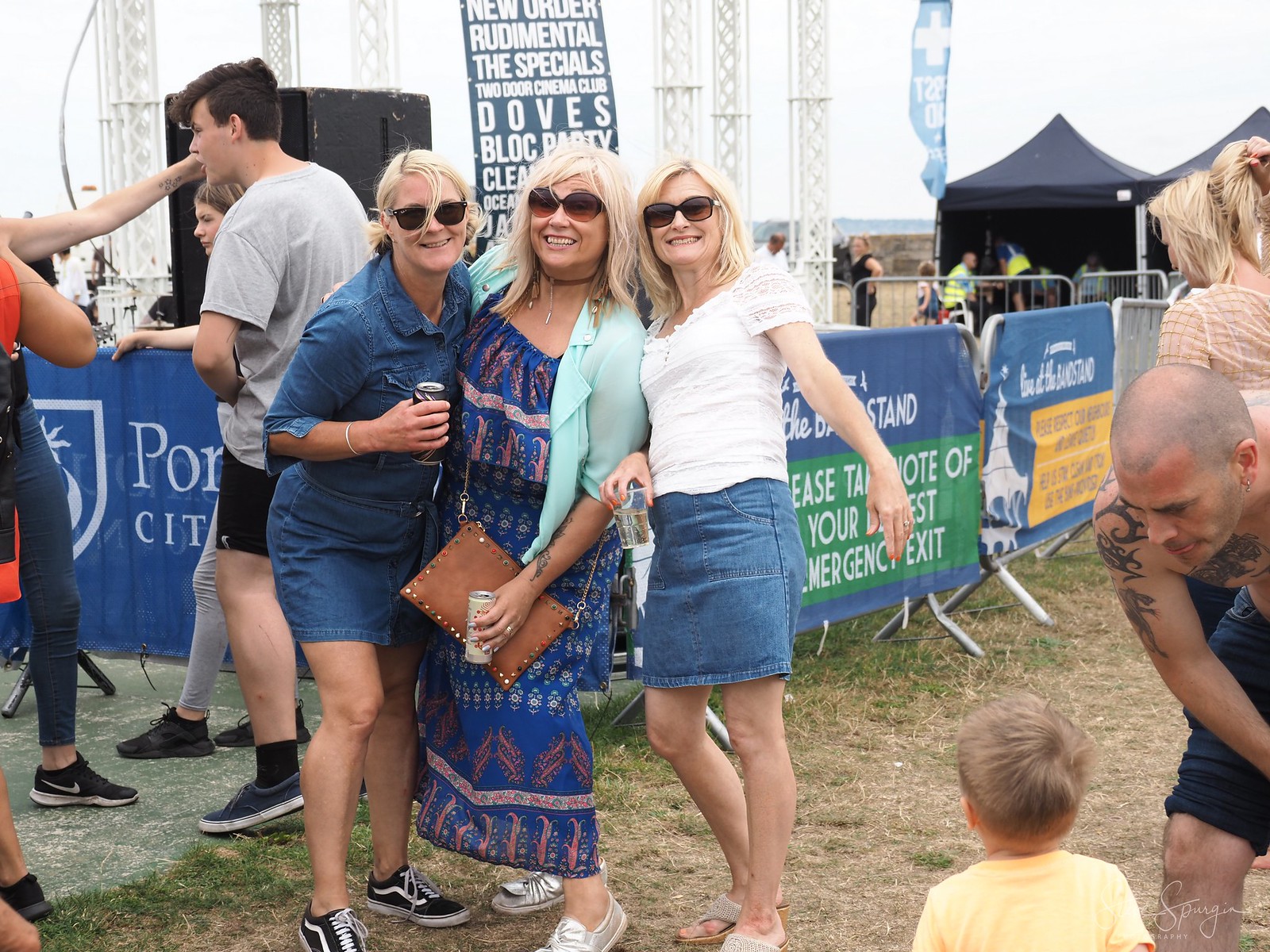A vibrant photograph captures the energy of an outdoor music festival on a sunny day. In the foreground, three middle-aged blonde women, all wearing dark sunglasses, pose cheerfully for the camera. On the left, one woman bends slightly, holding an open can in her right hand while wearing a blue denim dress and black-and-white sneakers. The lady in the middle, adorned in a full-length, blue and pink peasant-style dress, complements her look with silver sneakers. Leaning closely to her, the third woman sports a short-sleeved white blouse and a blue denim skirt, finishing her outfit with beige thong sandals.

Behind them stands a varied gathering; among them, a young blonde boy with his back to the camera gazes towards the women, and a tattooed, bald man with an earring is engaged nearby. The ground beneath them is a mix of grass and a concrete pad where a few young men stand.

In the background, festival signs and banners depict the names of bands like New Order, Rudimental, The Specials, Two Door Cinema Club, and Doves, indicating the event is likely a music festival. Further back, a blue and white First Aid banner with a red cross can be seen, and two tents, presumably housing EMTs, add a layer of safety to the festive atmosphere.